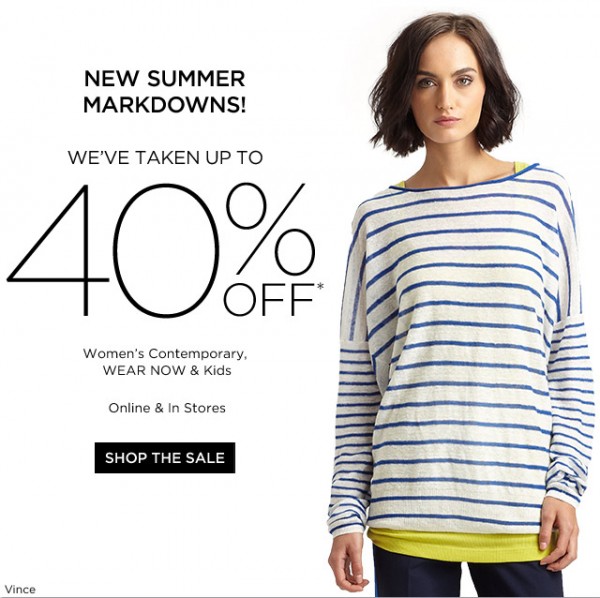Here's the detailed and cleaned-up caption:

---

**Ad Description:**

_Set against a white background, this advertisement prominently features bold black text slightly left of center declaring "New Summer Markdowns." Below it, in a lighter black font, it states "We've taken up to," followed by an eye-catching, oversized "40% off." An asterisk next to the discount hints at exclusions, suggesting the maximum discount is rarely applied. The text then lists categories: "Women's Contemporary, Wear Now, and Kids, Online and In Stores."

A black button with white text, "SHOP THE SALE!" in all caps and exclamation points, provides a call to action. In the lower left-hand corner, the word "Vince" appears mysteriously above a horizontal gray bar.

On the right-hand side of the ad, a striking woman gazes intently into the viewer’s eyes. She has neck-length brown hair stylishly parted to one side, with bold brown eyebrows and eyes accented by smoky makeup. Her lips sport a pale nude lipstick. She is dressed in a yellow undershirt overlaid by a white long-sleeve shirt with blue horizontal stripes, which change direction at the arms. The yellow undershirt peeks out from beneath the striped shirt. Completing the look, she wears blue pants (not jeans)._

---